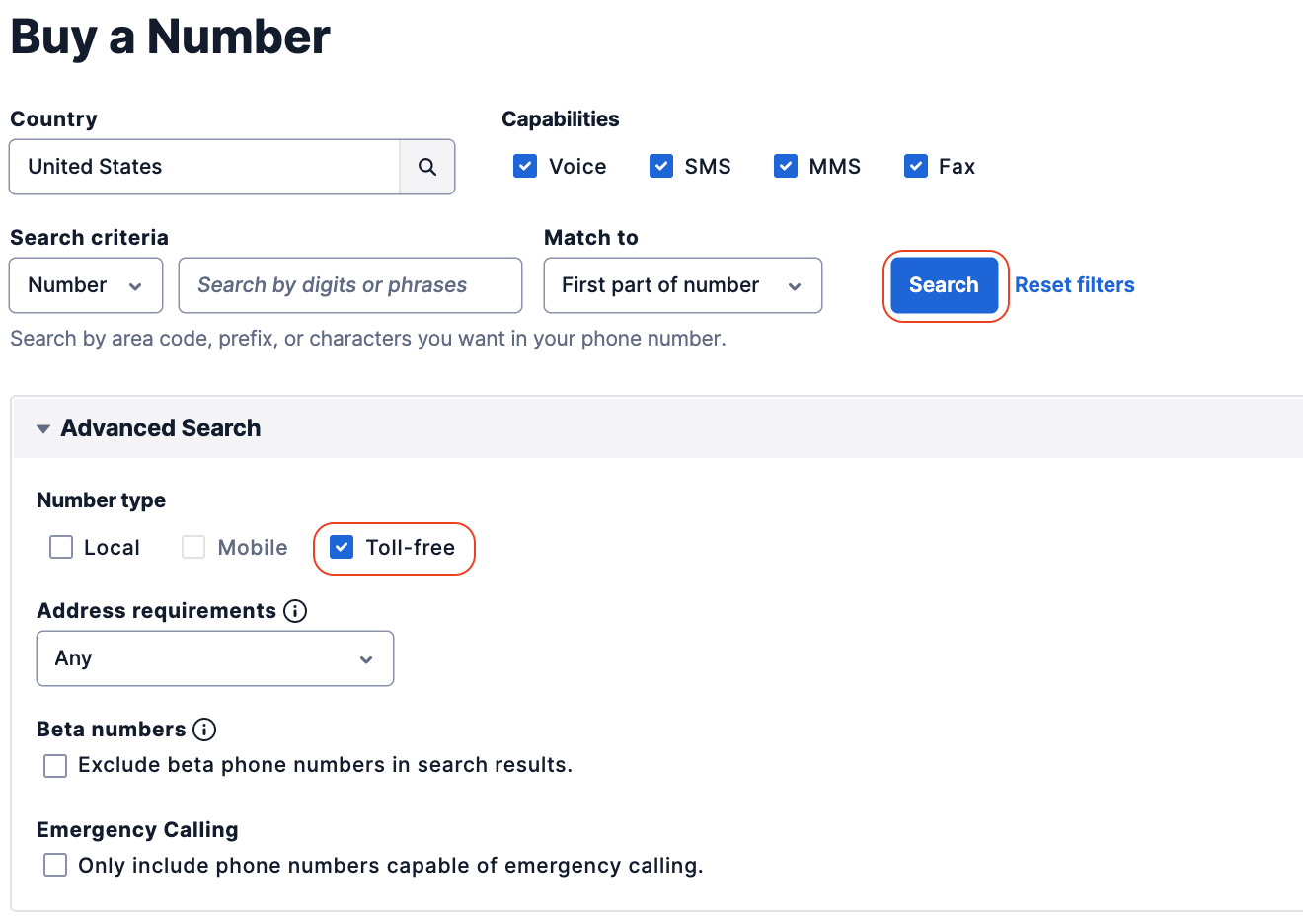**Caption:**

This screenshot captures a web page designed for phone number search and selection. At the very top, bold black text displays an unidentified number. Below, a dropdown menu labeled "Country" shows "United States" as the selected option. To the right, a section titled "Capabilities" lists four selectable features—Voice, SMS, MMS, and Fax—all marked with blue and white checkmarks indicating they are enabled.

Further down, the section "Search Criteria" features multiple input fields: one for entering a phone number, another for searching by digits or phrases, and another for specifying the first part of a number. Adjacent to these fields are a search bar and a "Reset Filters" button.

Continuing down, the text "Search by area code, prefix, or characters you want your phone number" is followed by an advanced search option. Under the "Number Type" section are three choices: Local, Mobile, and Toll-Free, with "Toll-Free" selected and highlighted with a red circle.

Next, the "Address Requirements" section includes a dropdown menu set to "Any". Beneath this, a small information icon (represented by a lowercase "i" inside a circle) is next to the phrase "Beta Numbers." An unchecked box labeled "Exclude beta phone numbers in search results" is displayed alongside it.

Finally, the last section labeled "Emergency Calling" asks if only phone numbers capable of emergency calling should be included, with the checkbox remaining unchecked.